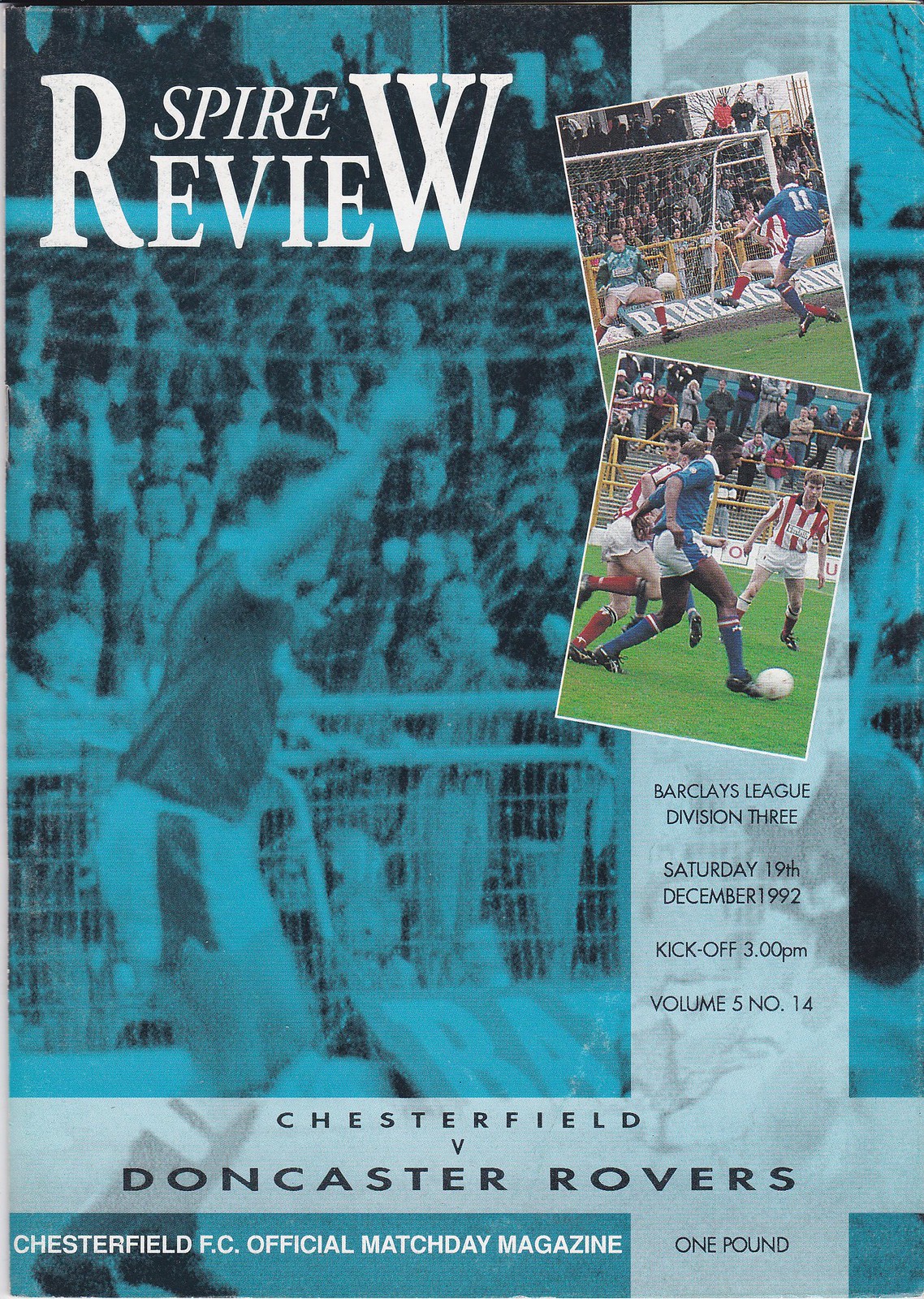The cover of the Chesterfield FC official match day magazine, titled "Spire Review," prominently features a blue and black design with a shadowy image of soccer players in the background, set against a lively audience. In bold white text, "Spire Review" stands out, with the R and W in "Review" extending tall and overlapping "Spear" at the top. To the side, two photographs are positioned: the first, slightly tilted left, captures a player kicking a soccer ball towards a goalie; the second, tilted right below the first, shows three players, including a black man in a blue uniform preparing to kick a soccer ball. Detailed text below the images indicates this is the Barclays League Division III match between Chesterfield and Doncaster Rovers, which took place on December 19, 1992, at 3 p.m., volume 5, number 14. The magazine is priced at one pound.